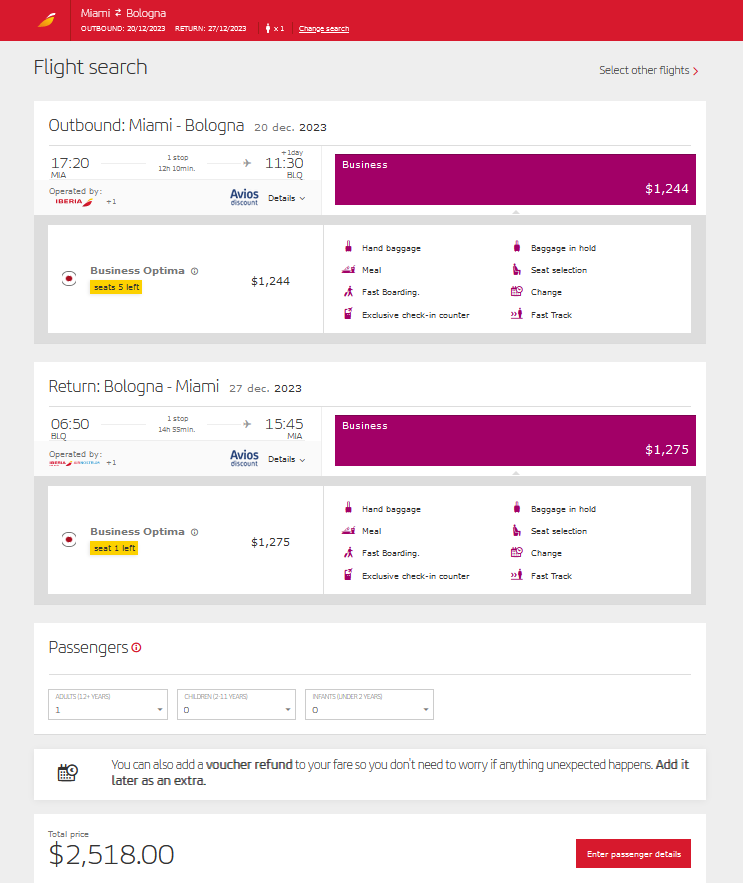The image appears to be a slightly blurry screen capture from a flight booking website, containing multiple sections laid out in a structured manner. 

At the top, a thin red banner features an orange and white feather-like logo, though the text is difficult to read due to the blurriness. Just below, a slightly blurry name is displayed, followed by three sections of white text underneath.

The main content of the page begins with a gray background hosting various windows. At the top, black text reads "Flight Search," and to the right, there is another black text section next to a red arrow that says "Select Other Flights."

The specific flight details are divided into several white boxes. The first box highlights the outbound flight from Miami to Bologna, dated 20th December 2023. This segment includes various colors of text: black, white, red, and blue fonts. The time of departure and arrival (17:20 to 11:30) and the relevant airport codes are also listed. Below this, there are logos of different sponsored companies, with a purple box to the side stating "Business 1244" in white font.

Scrolling down, the next window duplicated similar information but features a white background with black text and purple icons. The text reads "Business Optima," accompanied by a gold box that shows "5 Left" with a white circle and red dot. The price for this option is $1,244. Also listed are various perks, such as hand baggage, meal, fast boarding, checked baggage, the option to change the time, and fast track service. Each perk is represented by different icons including a cup, a person, food, and luggage.

The subsequent box provides information for the return flight from Bologna to Miami, scheduled for 27th December 2023. The departure and arrival times are 06:50 to 15:45, again with respective airport codes and the same purple and white box labeled "Business 1275." 

Recurrent options of "Business Optima" are shown with the same pricing and perks (hand baggage, meals, fast boarding, etc.) displayed with purple icons.

Moving further, a white box labeled "Passengers" includes three drop-down menus. Another white box with blackish text allows you to add a voucher refund to your fare, mentioned to cover unexpected occurrences, and can be added later as an extra service.

At the bottom, the total price of $2,518 is displayed in black text. Adjacent to this figure, a red button with white font is likely the final action button for booking.